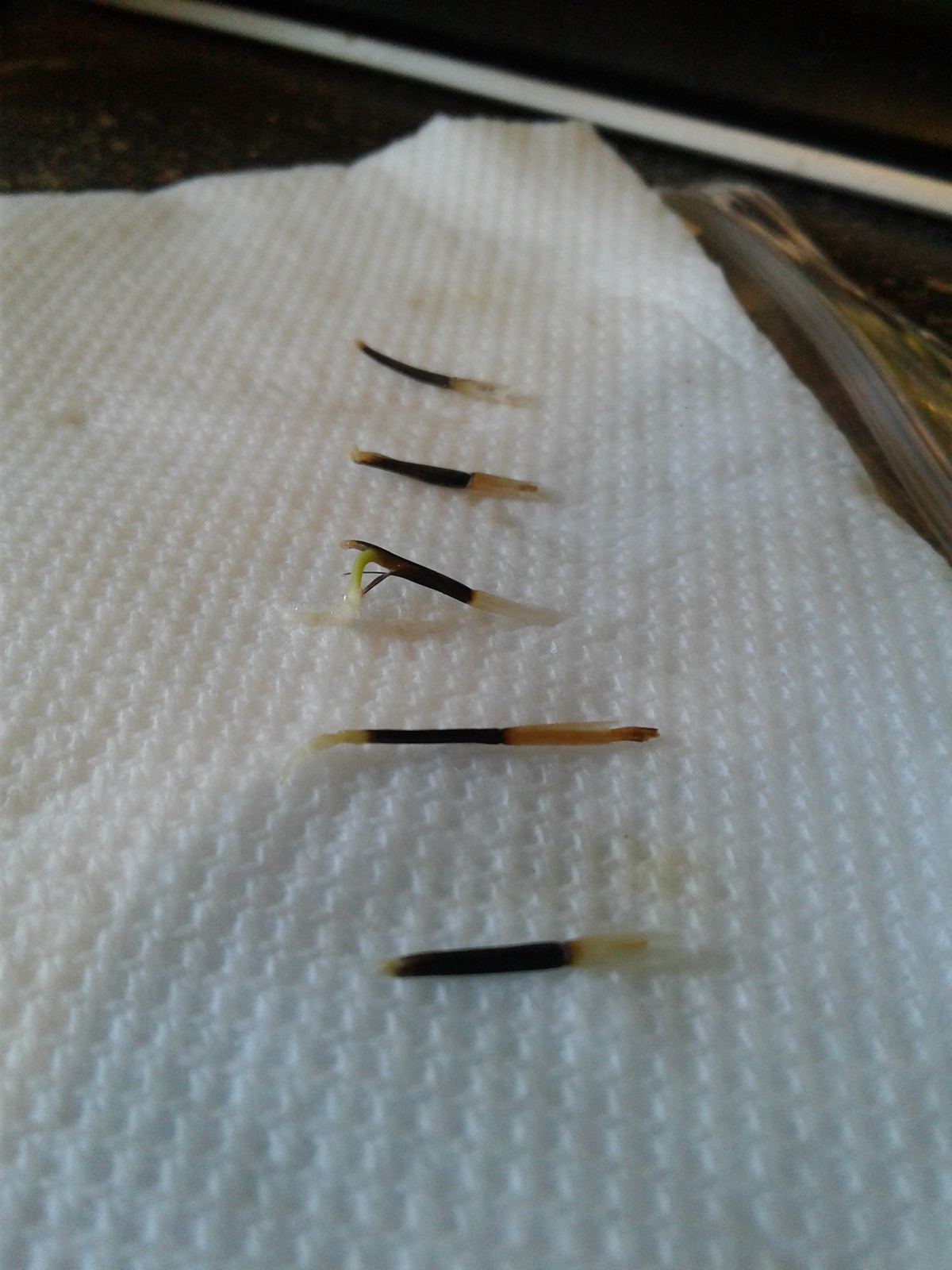This is a detailed color photograph capturing a vertical arrangement of five thin objects resembling semi-burnt-out matches or seed pods. These horizontally aligned objects display a gradient from green edges to a black central band, ending in a yellow or tan color. They are positioned on a crumpled, texturized white paper towel or napkin, which seems to have absorbed some stain from the objects. The napkin forms a triangular shape towards the top middle of the image. The top of the photograph is dominated by a black background, intersected by a diagonal white line. To the far right, partially obscured behind the napkin, is a grey object with yellow and black edges, possibly suggesting another layer or item beneath the main scene. In the top right corner, faintly visible, is part of a brown and black polka-dotted table. The entire arrangement rests on what appears to be a clear ziplock bag.